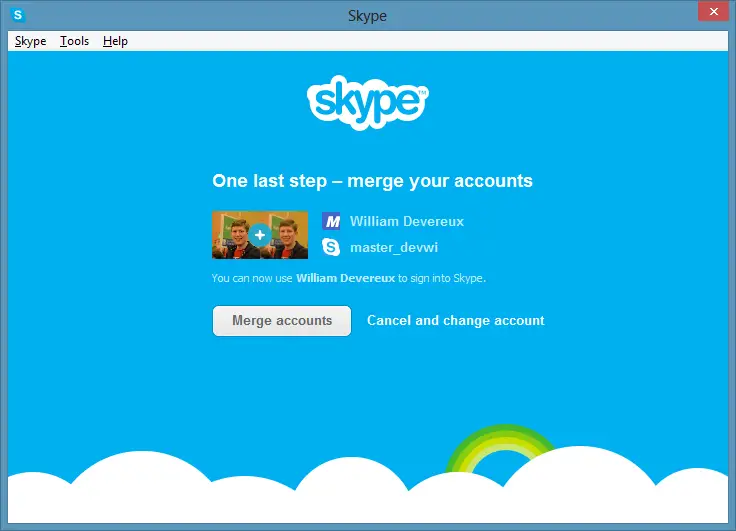The image features a visually intricate Skype interface. The background consists of a large blue rectangle. At the top right is a lighter blue square with an "S" in it, symbolizing Skype. In black text, the word "Skype" is prominently displayed below the square. Adjacent to it, on the right-hand side, is a red rectangle with an "X" inside, likely serving as a close button.

Beneath these elements, there's a white rectangle displaying "Skype, Tools, and Help" in text. Further down, a light blue rectangle contains cloud-like patterns at the bottom. Nestled within these clouds are a blue circle, a yellow circle, and a green circle, partially obscured by the cloud imagery.

At the top center of this section, the Skype logo appears, heavily outlined in white, spelling out "Skype." Below the logo, the text "One Last Step – Merge Your Accounts" is prominently displayed. A picture of two men is shown with a blue circle containing a plus sign between them, suggesting a merging action.

Toward the bottom right, a purple square with a white "M" inside appears next to the name "William Devereux" spelled out clearly. Nearby, there is a cloud icon with an "S" in it, labeled "Master_DEVWI," indicating another account or username. The message states that William Devereux can now use this account to sign into Skype.

At the bottom, there's a white rectangle with curved corners, featuring the text "Merge Accounts." Below that, a partially visible blue rectangle merges into the blue background, containing the options "Cancel" and "Change Account."